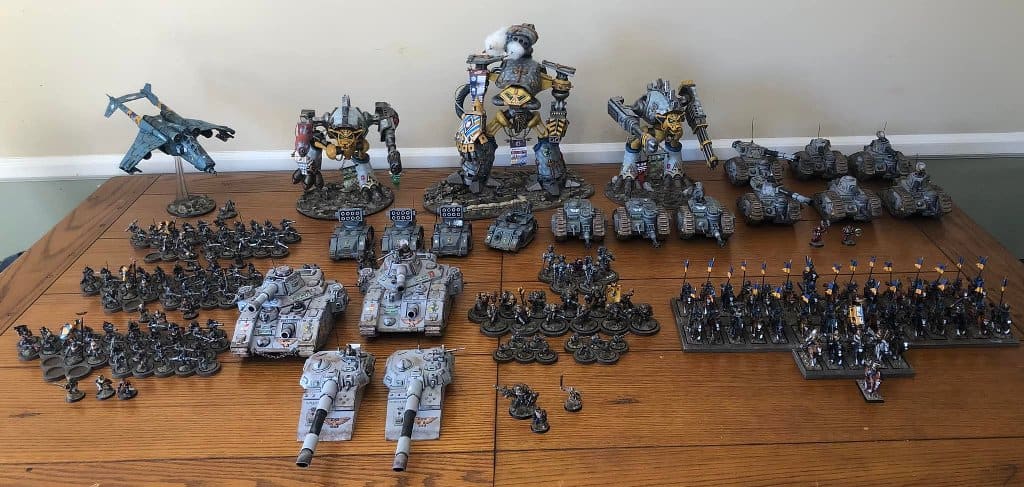The photograph showcases an elaborate arrangement of meticulously crafted, die-cast sci-fi toys displayed on a brownish wooden table against a light cream or tan backdrop. In the foreground, several larger, light gray tanks are positioned on the left, while darker gray tanks and armored personnel carriers are placed towards the right. Dominating the scene are three large robotic figures resembling Transformers, primarily gray with touches of yellow and orange, towering towards the center-top of the image. Among these robots are an array of approximately 10 to 12 smaller tanks aligned towards the back and right. On the upper left side of the image, a greenish jet fighter is mounted on a stand, angled downwards. Additionally, scattered human figurines and possible motorcycles or mounted figures appear particularly on the left and front right of the scene, enhancing the intricate tableau of this sci-fi toy collection.